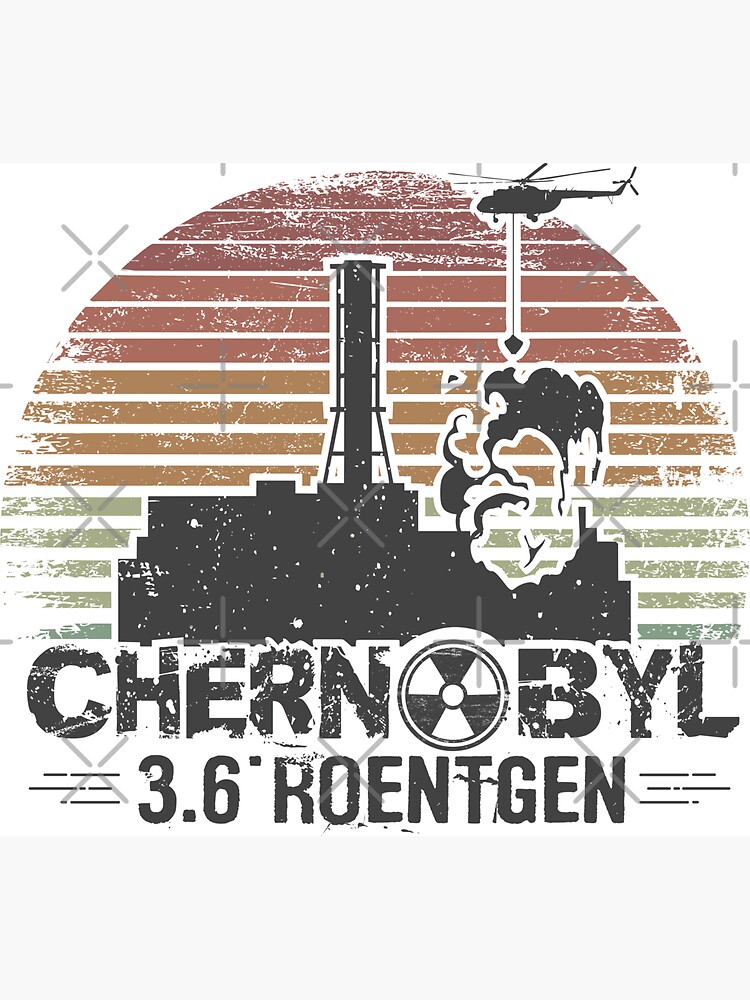This is a detailed graphic design depicting the Chernobyl nuclear accident. Central to the illustration is the Chernobyl power plant, which appears to have just exploded, emitting thick smoke. A firefighting helicopter hovers above the right side of the building, lowering a bucket via a rope into the smoky area of the explosion. Dominating the scene is a large smokestack standing tall amidst the industrial chaos. The name "Chernobyl" is prominently displayed in big, black, distressed lettering beneath the building, with the O cleverly replaced by a radioactive symbol. This is complemented by the text "3.6 roentgen" beneath it, referencing the level of radiation. The background features a stylized, gradient design resembling a sun, rendered in horizontal stripes of dark green, rust, tan, orange-brown, and reddish-brown tones, contributing to a duotone effect. The entire graphic has a deliberately worn and weathered look, enhancing the historical and catastrophic feel of the depicted scene.